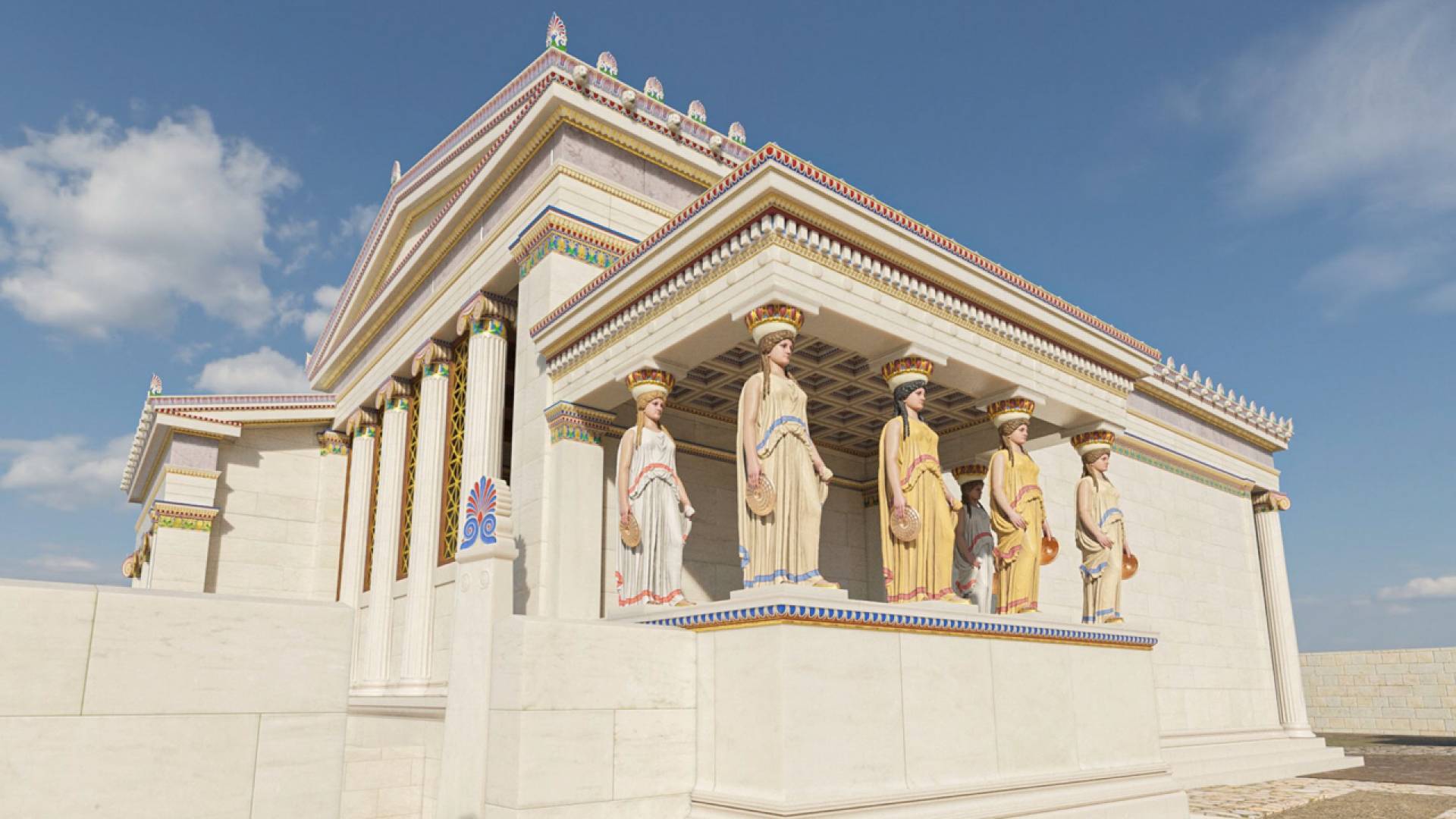This horizontally-oriented digital illustration depicts a meticulously detailed and well-preserved Greek or Roman temple replica, possibly situated outside of Greece or Rome. The cream-colored, two-story structure showcases a series of traditional fluted columns on the left side and an adorned front portico held up by five intricately designed female statues, with an additional partially visible statue. These statues, clad in richly colored toga gowns featuring whites, yellows, blues, reds, and browns, support the porch roof with their crowned heads. The building is adorned with elaborate molding and ornate features that mirror the vibrant colors of the female figures' attire. The light beige marble-like material of the temple stands against a backdrop of a medium blue sky filled with a mix of puffy and wisp-like clouds. The corners of the building are intricately detailed, with the nearest corner featuring inset statues and designed ceilings, enhancing the overall grandeur and authenticity of this replica temple.